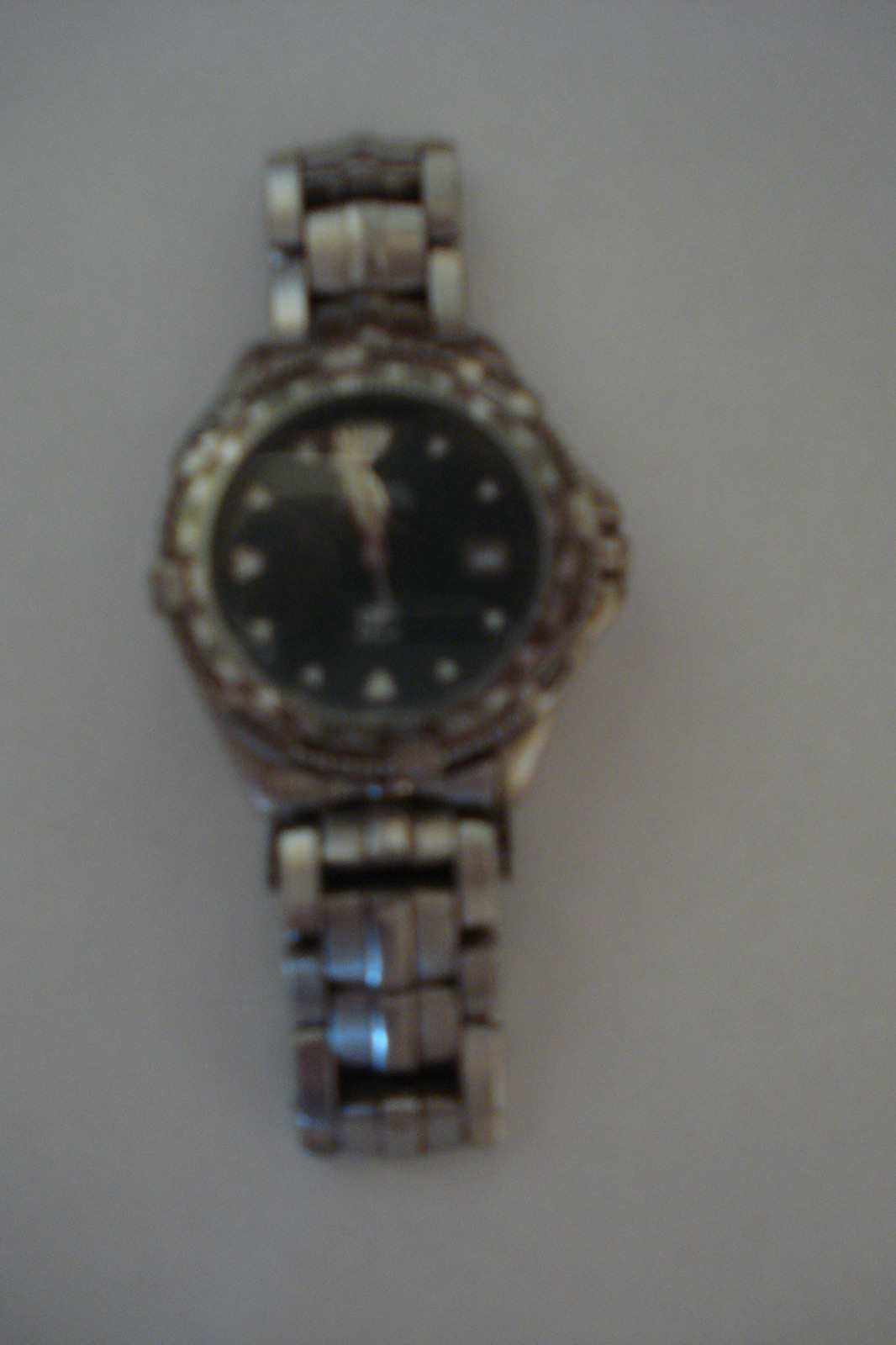This is a somewhat blurry photograph of a silver metal watch, lying face up on a white background and illuminated by overhead lights, resulting in some reflections on its surface. The watch features a chain of silver links and a silver bezel encircling its dark blue face, which appears black in dim lighting. The watch face lacks numbers, instead using various markers: large silver triangles at the 12, 6, and 9 positions, and a small white square at the 3 o'clock position, typically indicating a date window. The silver hands stand out against the dark face. To the right is a recessed silver dial, likely for adjusting both the date and time. Despite the blurriness of the image, the overall design and details of the watch suggest a sophisticated style, potentially with additional decorative elements around the face.